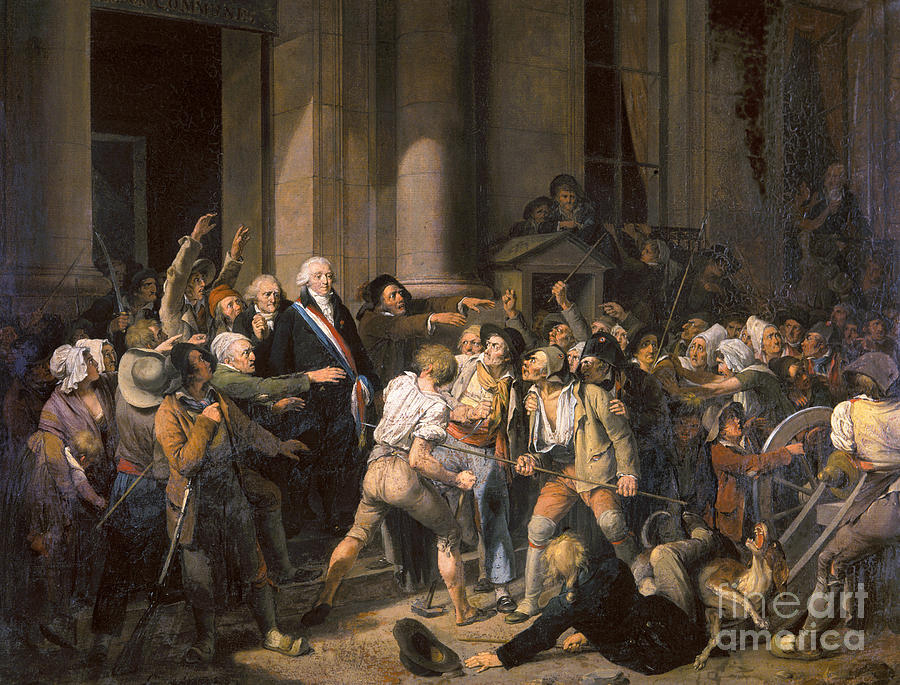The image is a historical painting, likely from the colonial era, depicting a chaotic scene with significant detail and emotional intensity. It features a central figure who appears to be George Washington or another prominent historical figure from that time period, distinguished by his white, fluffy wig and a suit adorned with a red, white, and blue sash. He stands on a set of steps, surrounded by a horde of distressed and agitated people dressed in tattered, peasant-like colonial clothing. In the bottom right corner, the painting is marked with a Fine Art America watermark. The scene is filled with tension, as people brandish sticks and swords, shout, and reach out with angry and scared expressions. Notably, one man holding a long fire poker stares up at the central figure with fury, while another has fallen to the ground, losing his black hat in the process. There is also a distressed dog being pushed over amidst the turmoil. The edges of the painting show signs of age, with visible cracking and fading, adding to its historical atmosphere.